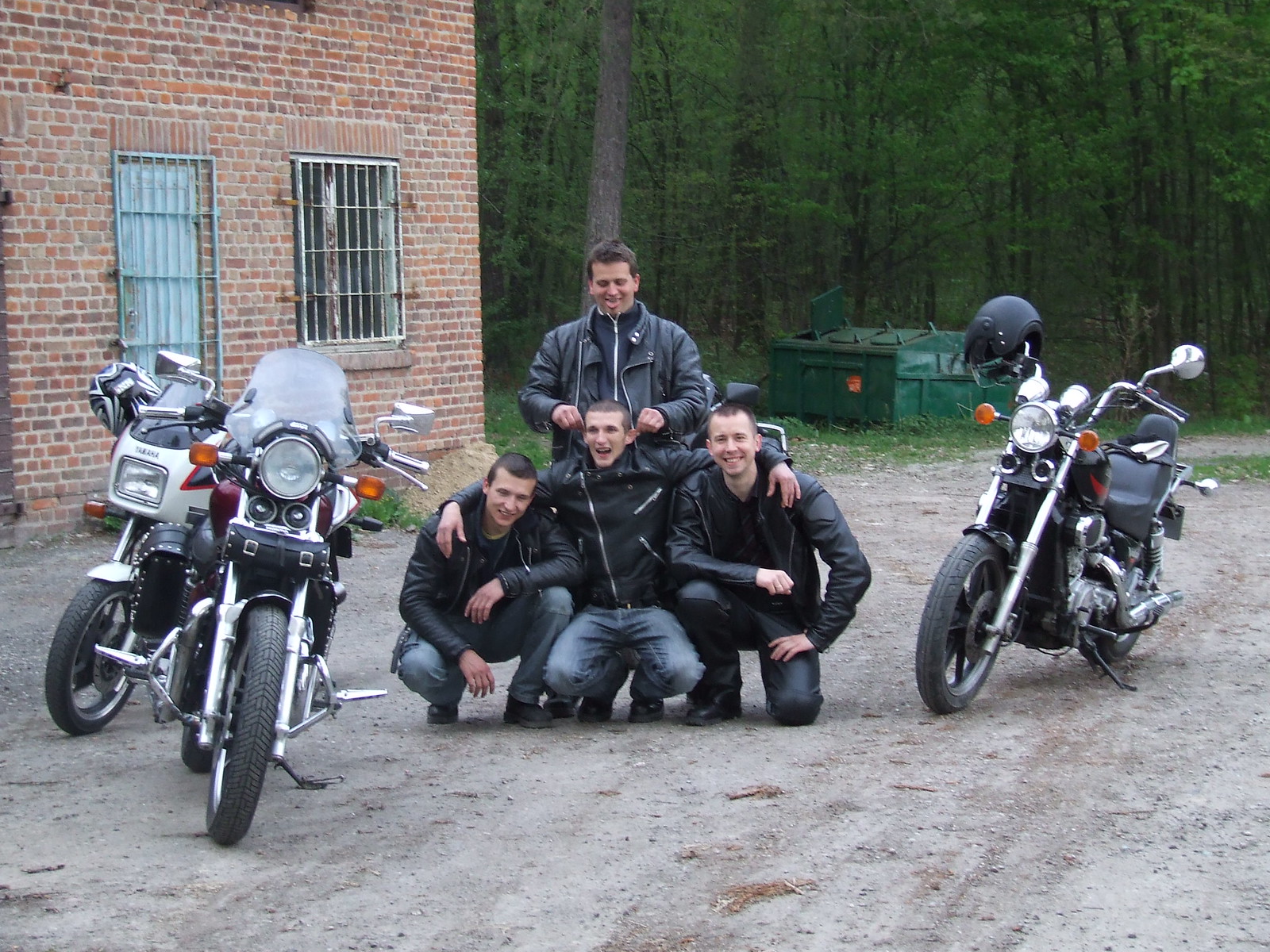This outdoor photograph, taken on the edge of a forest, features a red brick building with metal bars over the windows and a green metal bar on the door. Nearby, there's a green structure and a dumpster. The foreground reveals a dirt and gravel driveway with four motorcycles, two of which have helmets hanging from their handlebars. Four men, all dressed in blue jeans and black leather biker jackets, are gathered around the motorcycles. Three of them are crouched down with their arms around each other, while the fourth man stands behind the center crouching man, playfully lifting his ears. All four men are smiling and laughing, with the man in the back even sticking out his tongue, creating a lively and spirited group photo.